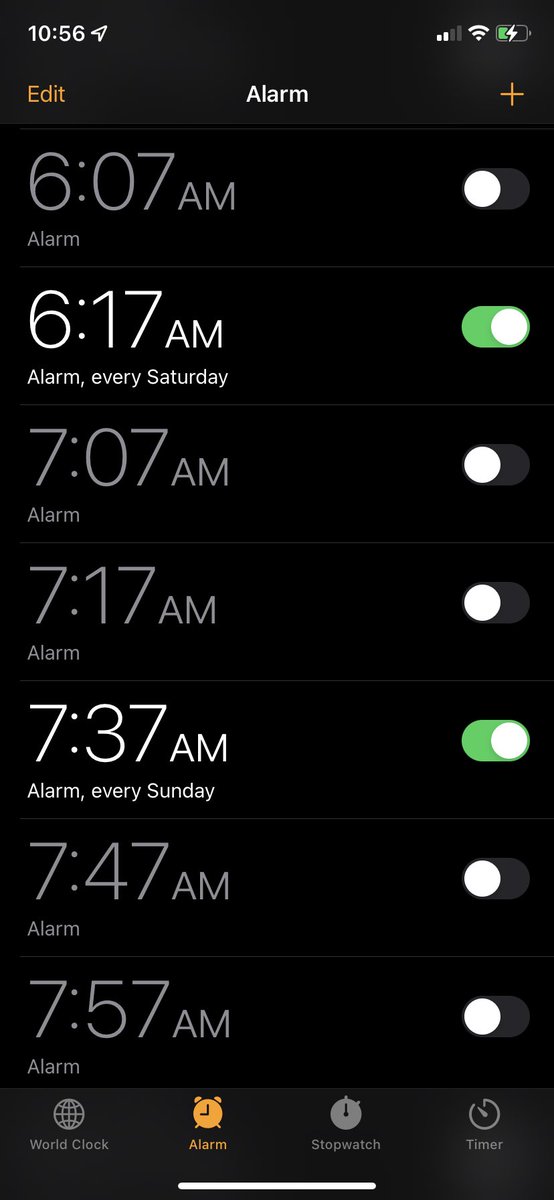This image is a screenshot from an iPhone, displaying the Alarm section within the Clock app. The screen has a black background, drawing focus to various detailed elements at the top and throughout the screen.

At the top left corner, the time is displayed in white as "10:56" with a small navigation arrow beside it. On the right side of the top header, there are icons indicating the phone's status: a partially filled cell signal icon with two white bars and two gray bars, a fully lit Wi-Fi signal icon, and a battery icon showing a lightning bolt in the center. The left side of this battery icon is green, indicating charging, and the right side is black.

Below the status bar, three text elements are aligned from left to right: "EDIT" in an orangey-yellow, "ALARM" in white, and a plus (+) sign also in the orangey-yellow color. A faint line divides this header from the main content of the screen.

The main section lists seven alarms, each displayed horizontally with a toggle switch on the right:

1. **6:07 AM** - Marked as "ALARM" underneath the time in light gray. The toggle switch is off, indicated by a white circle on the left and a dark gray background.
   
2. **6:17 AM** - Marked as "ALARM, every Saturday" underneath the time in bright white font. The toggle switch is on, with a bright green background and a white circle on the right.

3. **7:07 AM** - Marked as "ALARM" in light gray, with the toggle switch off (white circle on the left, dark gray background).

4. **7:17 AM** - Similarly marked as "ALARM" in light gray, the toggle switch is off.

5. **7:37 AM** - Marked as "ALARM, every Sunday" in bright white font, with the toggle switch on (bright green background, white circle on the right).

6. **7:47 AM** - Marked as "ALARM" in light gray, with the toggle switch off.

7. **7:57 AM** - Also marked as "ALARM" in light gray, with the toggle switch off.

The footer of the screen includes four icons aligned horizontally. From left to right:

- A globe icon labeled "World Clock".
- An alarm clock icon labeled "ALARM" in the same orangey-yellow color.
- A stopwatch icon labeled "Stopwatch" in gray.
- A timer icon labeled "Timer" in light gray.

These icons provide navigation within the Clock app, offering quick access to different functionalities.